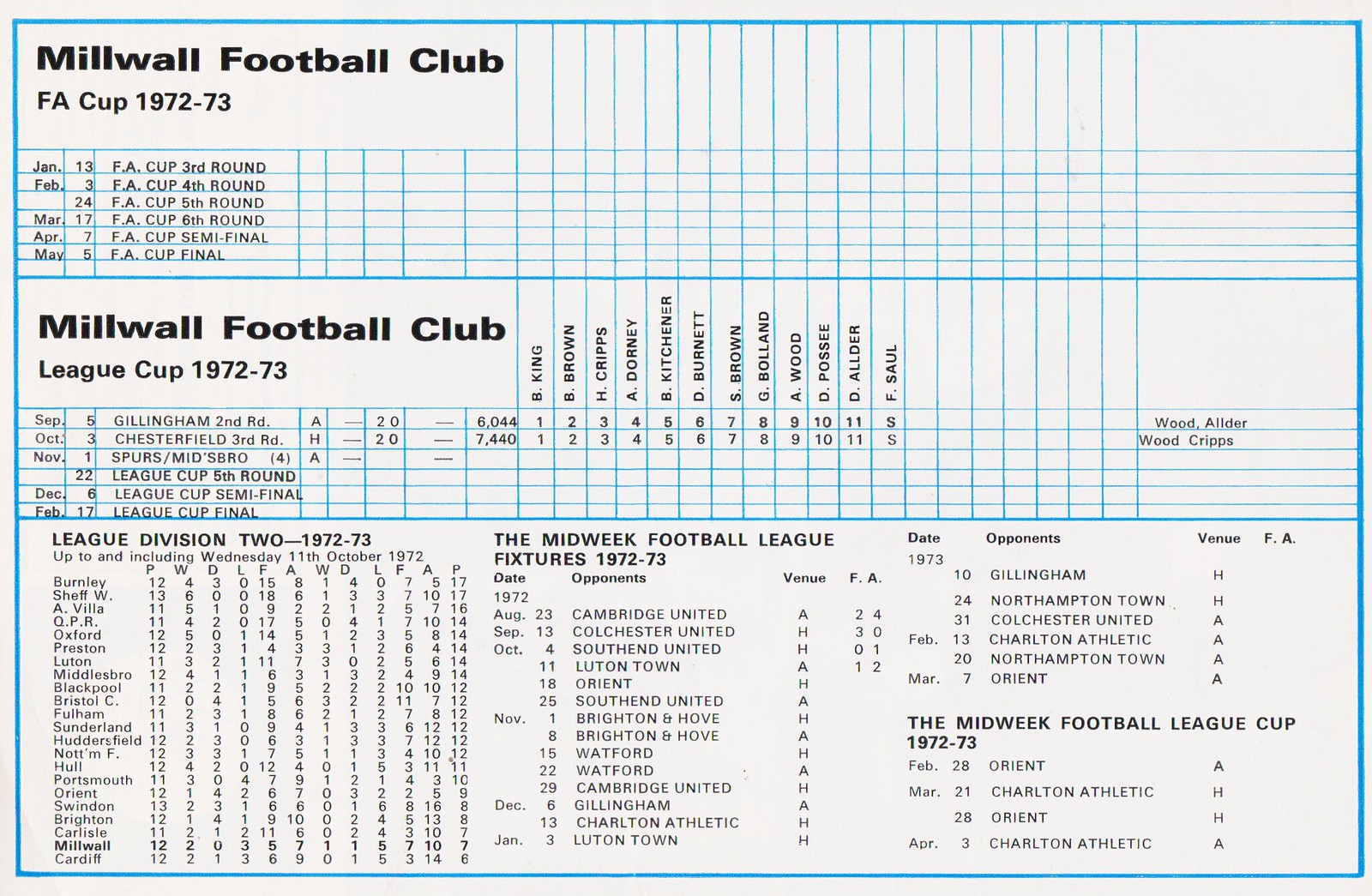The image is a scan of a paper document containing multiple tables with detailed soccer statistics and schedules for the Millwall Football Club during the 1972-1973 season. It predominantly features a blue grid on a white background. The top left section is titled "Millwall Football Club FA Cup 1972 to 73," listing dates from January to May followed by rounds of the FA Cup, from the third round to the final. Directly below this is another section for the "Millwall Football Club League Cup 1972 to 73," detailing dates from September to February with corresponding cup rounds and opponents.

At the center of the image, there is a table with six names, presumably player names—B. King, B. Brown, H. Cripps, A. Dorney, B. Kitchener, and B. Durnett—accompanied by numbers. Surrounding these central details are columns and lists showing league performances, including "League Division II 1972-73" with win-loss records for various teams, and "Midweek Football League Fixtures 1972 to 73," outlining specific match dates, venues, and opponents.

The right side features another section for matches, showing date, opponents, and venues, indicating whether it was a home or away game. The "Midweek Football League Cup 1972-73" section at the bottom right includes three dates, opponents, and venue details. Overall, the tables and sections comprehensively outline the fixtures, player statistics, and performance metrics for the Millwall Football Club in multiple competitions during the 1972-1973 season.